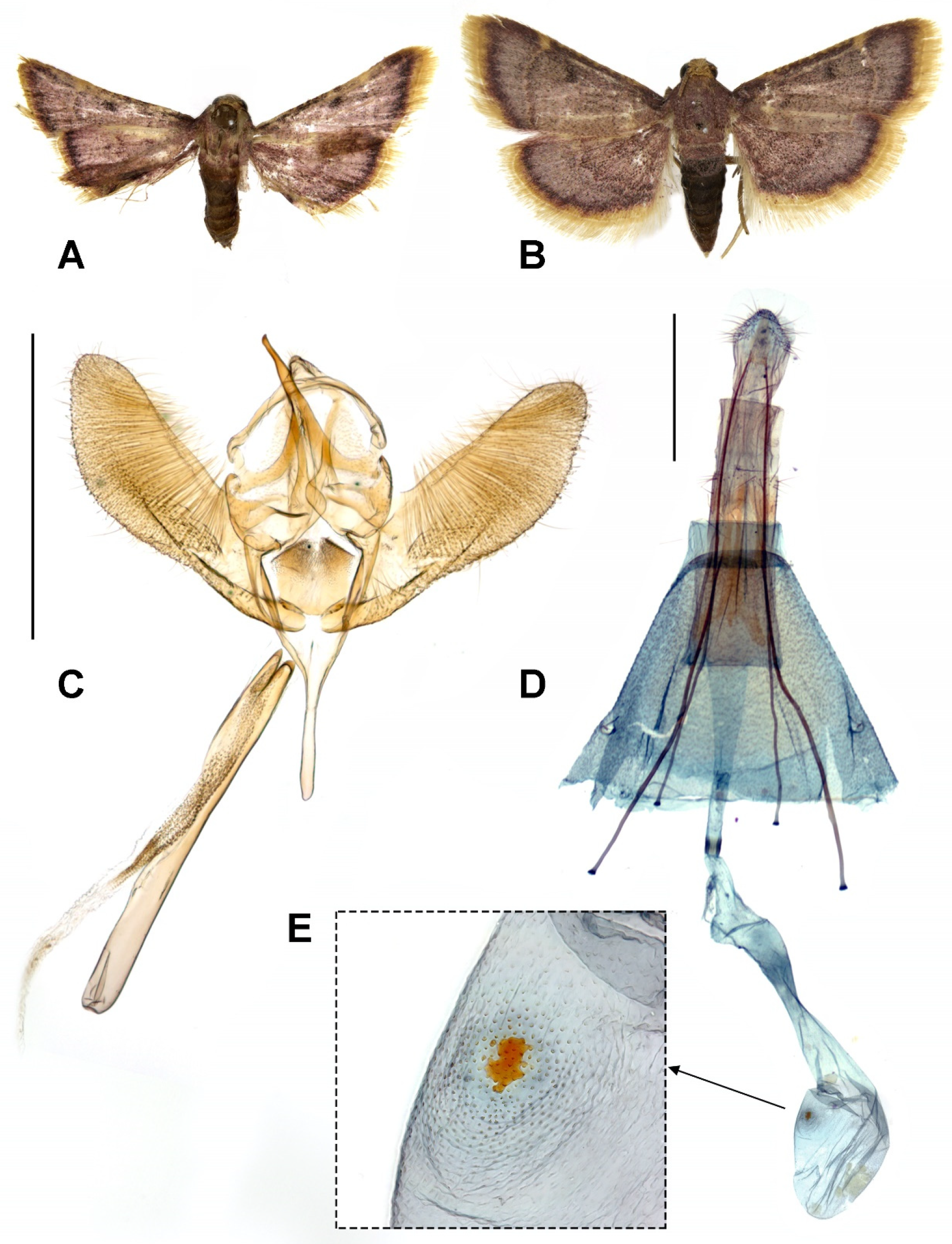This scientific image showcases five diagrams of moths, each labeled from A to E. In the top left corner, Diagram A features a brown moth, followed by Diagram B which depicts a larger brown moth of similar appearance. At the center, Diagram C illustrates a golden-colored, detailed diagram of the moth and its wings, emphasizing the intricate structure. To its right, Diagram D presents a see-through, x-ray-like image of a moth wing, revealing its detailed vein structure. Finally, at the bottom center, Diagram E provides a close-up view of a section of the moth's wing, highlighting the texture and patterns in a square frame.